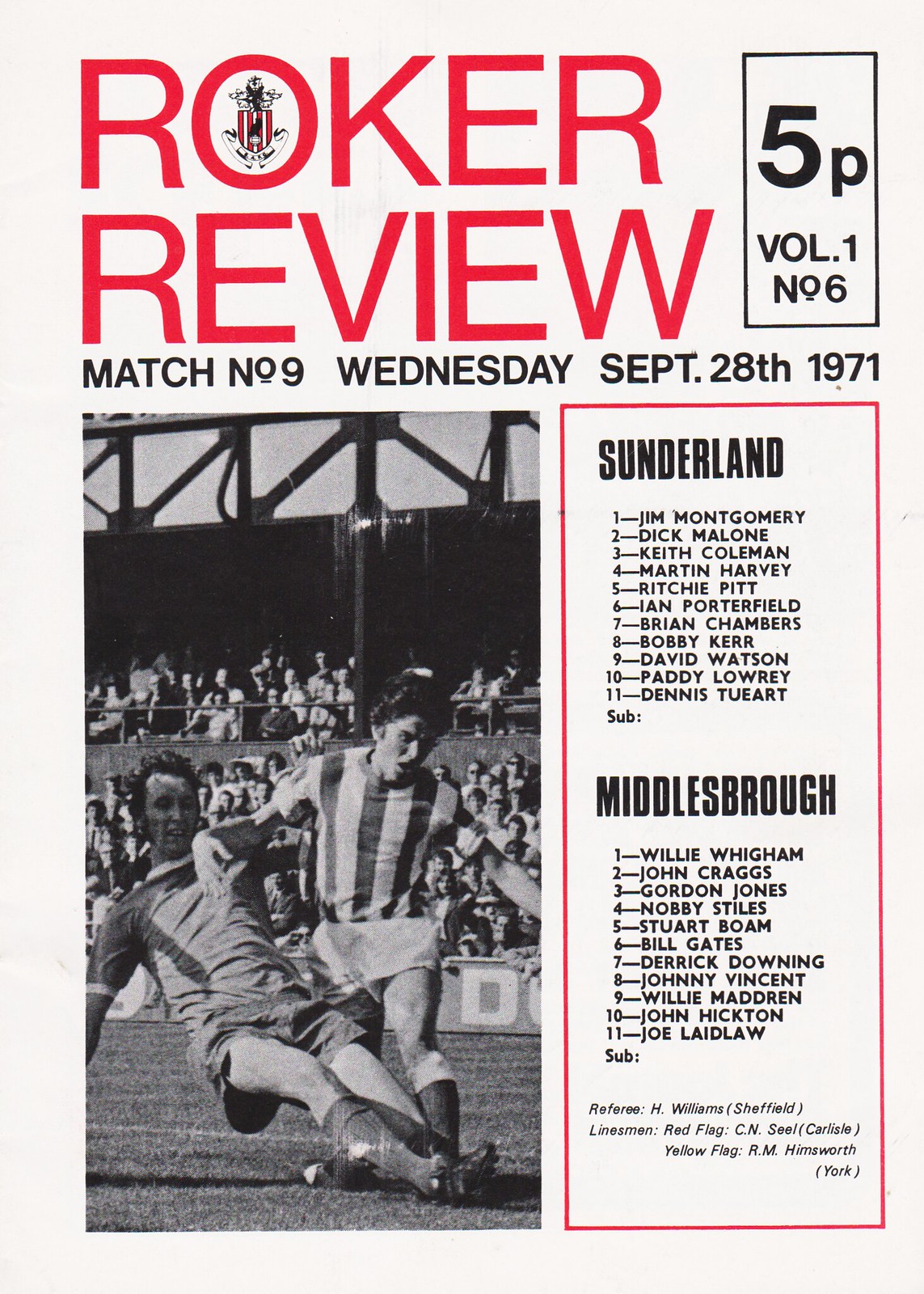Front page of the "Roker Review" magazine, dated Wednesday, September 28, 1971, boldly displayed in red font at the top left corner. The edition details read "5P Volume 1 Number 6 Match Number 9" in black font. A vintage black-and-white photograph at the bottom left features a dynamic soccer scene where a player in a solid-colored shirt is falling while another in a striped jersey moves to intercept. To the right of the image, under a red square box titled "Southern Wind," are the names of the Sunderland team players: Jim Montgomery, Dick Malone, Keith Coleman, Martin Harvey, Richie Pitt, Ian Porterfield, Brian Chambers, Bobby Kerr, David Watson, Patti Loray, and Dennis Tueart, with "sub" mentioned but left blank. The opposing team is Middlesbrough, with players listed as Willie Ligham, John Craggs, Jordan Jones, Nobby Stiles, Stuart Baum, Bill Gates, Derrick Downing, Johnny Benson, Willie Madren, John Hickton, Joe Labol, and "sub." Match officials included Referee J. H. Williams from Sheffield and Linesmen identified by flags, though finer details are obscured.